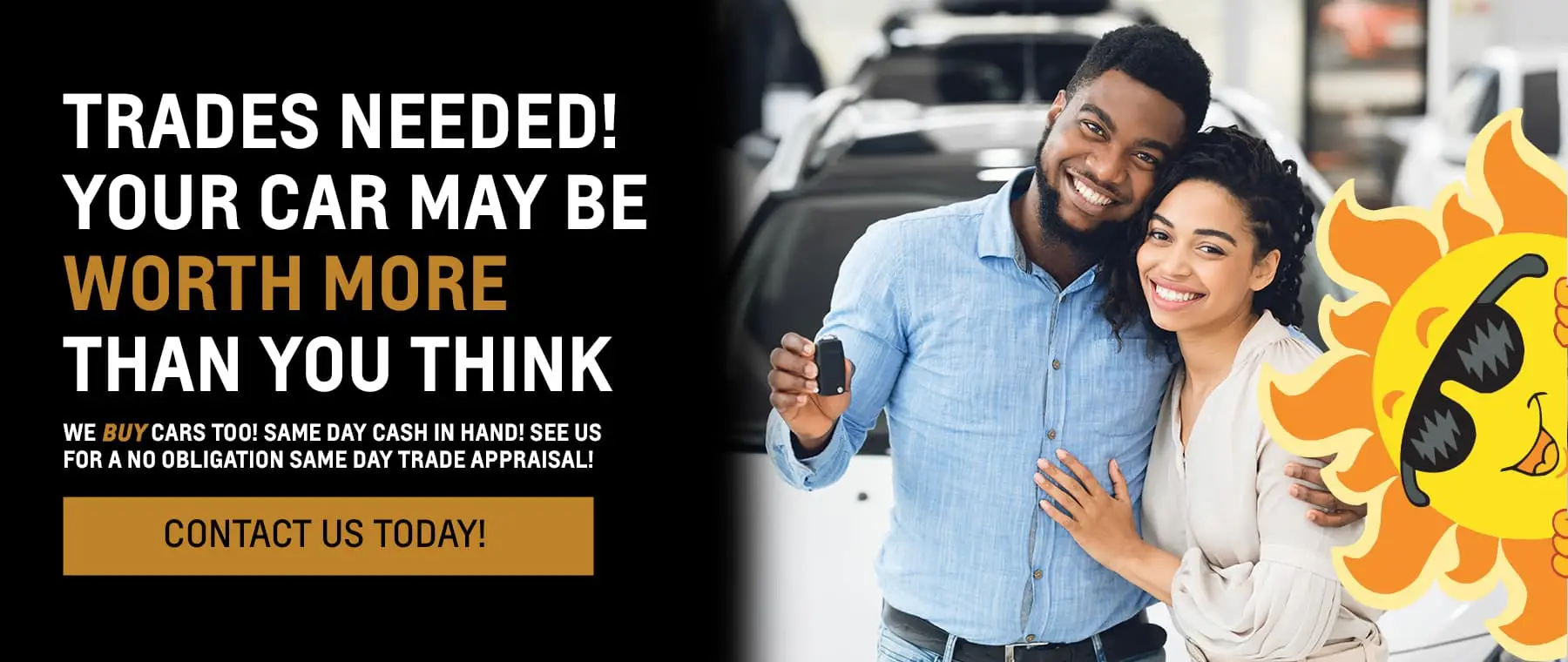The advertisement is displayed in a narrow, landscape format. On the left side, a black background hosts bold white text declaring, "TRADES NEEDED!" in large uppercase letters. Following in smaller white uppercase text, it reads, "YOUR CAR MAY BE," then switches to burnt orange on the next line with "WORTH MORE," and concludes with, "THAN YOU THINK." Beneath this, in very small white uppercase letters, it states, "WE BUY CARS TO SAME DAY CASH IN HAND, SEE US FOR A NO OBLIGATION SAME DAY TRADE APPRAISAL," with the word "BUY" highlighted in burnt orange. Below this message, an orange block displays "CONTACT US TODAY" in black.

To the right, the image seamlessly transitions from the black background into a photograph. The photo features a joyful Black couple holding car keys, surrounded by several vehicles, suggesting a successful transaction. The man, located near the center, wears a blue shirt and what appears to be denim pants. Beside him, the woman, positioned to the right of the image, dons a cream long-sleeve blouse with her hair stylishly pinned up on one side. She is not seen wearing a wedding ring, and the man’s left hand is not visible.

On the far right side, adding a playful touch, a cartoon sun donning sunglasses peeks into the picture, emitting bright orange rays around its yellow core, contributing a cheerful and inviting atmosphere to the ad.